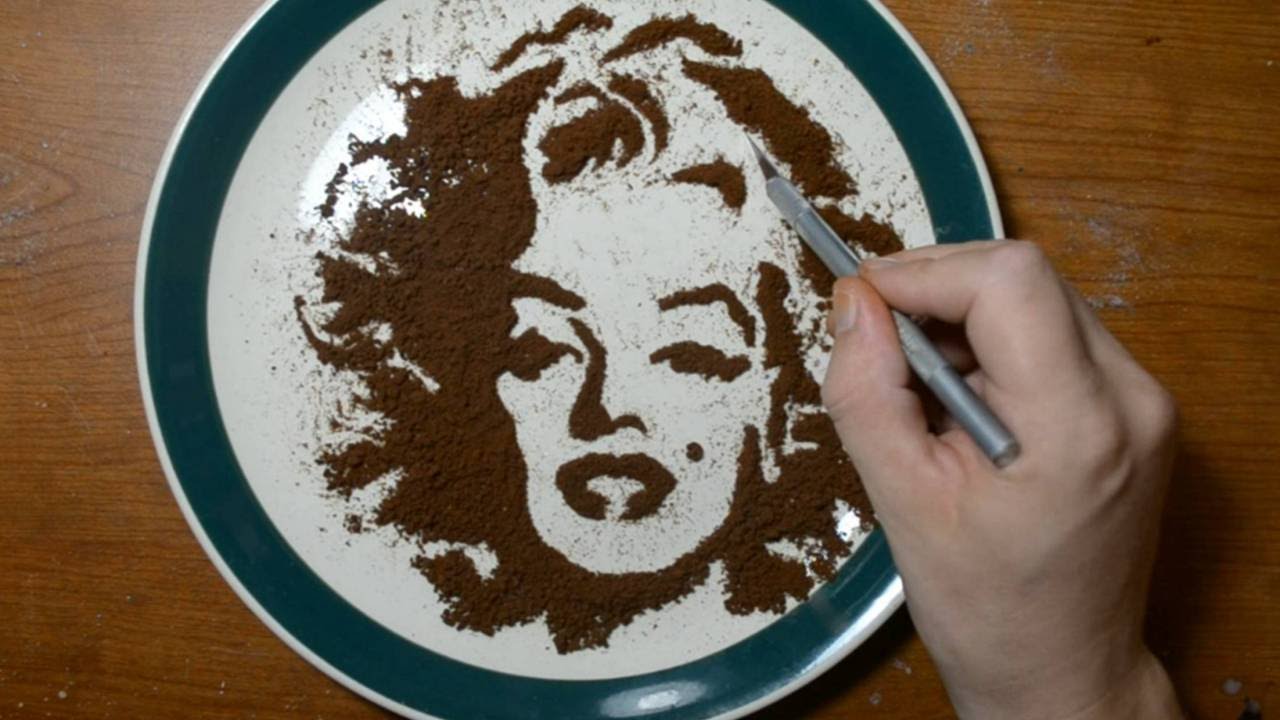The image depicts a close-up view of a white plate with a dark blue rim, placed on a reddish-brown wooden table. At the center of the plate, an artist is intricately crafting the face of Marilyn Monroe using coffee grounds. The artist's hand, holding an X-Acto knife, is visible, indicating they are in the process of finely detailing the iconic features of Monroe, including her famous mole, distinctive lips, and expressive eyes. The coffee grounds are carefully shaped to create a striking contrast with the white background of the plate, making Marilyn's face vividly clear. The photograph is taken from above and is notably well-lit, likely due to natural lighting, enhancing the clarity and detail of the artistic process.